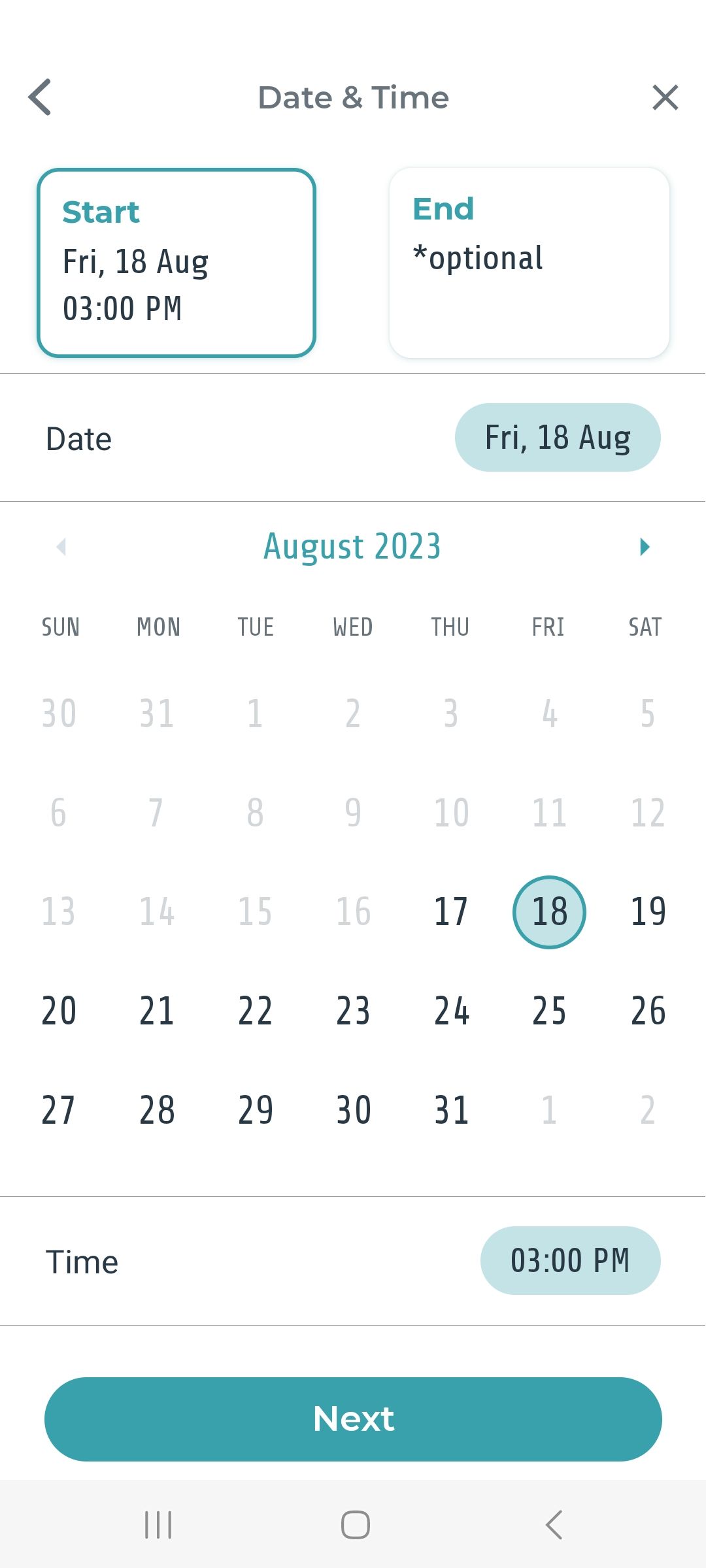This screenshot from a calendar app on an Android device features an interface designed for scheduling events. The bottom section displays the typical Android navigation buttons: three vertical dots on the left, a white square with a gray outline in the middle, and a left-facing arrow on the right for navigation. At the top, the all-white background of the app contrasts with the light gray text and icons.

In the top-left corner, there is a left-facing arrow icon for going back. Centrally positioned at the top, the words "Date and time" are rendered in light gray text. The top-right corner houses a light gray 'X' button for closing the screen.

Just below these top elements, a turquoise-outlined white box provides the Start date and time details: "Friday, Aug 18, 3:00 PM." Adjacent to this on the right is a white button labeled "End (Optional)" with a star icon next to the word "Optional."

Further down, the calendar for August 2023 is displayed, showing that Friday, August 18th, is currently selected. This date is marked with a bluish outline circle. Dates from July 30th through August 16th are grayed out, indicating they are not selectable, suggesting that today is probably August 17th.

Below the calendar, the selected time is indicated as 3:00 PM. At the bottom of the screen, a blue ‘Next’ button is available for proceeding to the next step in the scheduling process.